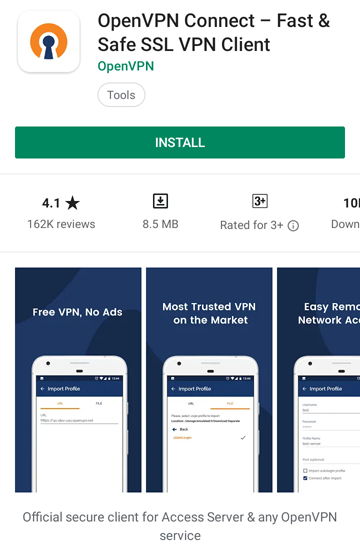The screenshot depicts an application interface for a Safe SSL VPN client. The primary icon is shaped like a keyhole, representing security. The app, identifiable by its green triangle logo, highlights compatibility with OpenVPN. The interface shows the app's rating as 4.1 stars from 162,000 reviews. The app is 8.5 MB in size and rated suitable for ages 3 and up. Three rectangular sections provide additional context, each displaying a picture of a mobile phone. The first rectangle emphasizes "Free VPN, No Ads," suggesting it's the most trusted VPN on the market. The third rectangle, partially cut off, seems to highlight easy remote network access with phrases such as "easy remote" and possibly "REM." At the bottom, it states, "Official secure client for Access Server and any OpenVPN service," indicating its official capacity. The background of the screenshot is white.